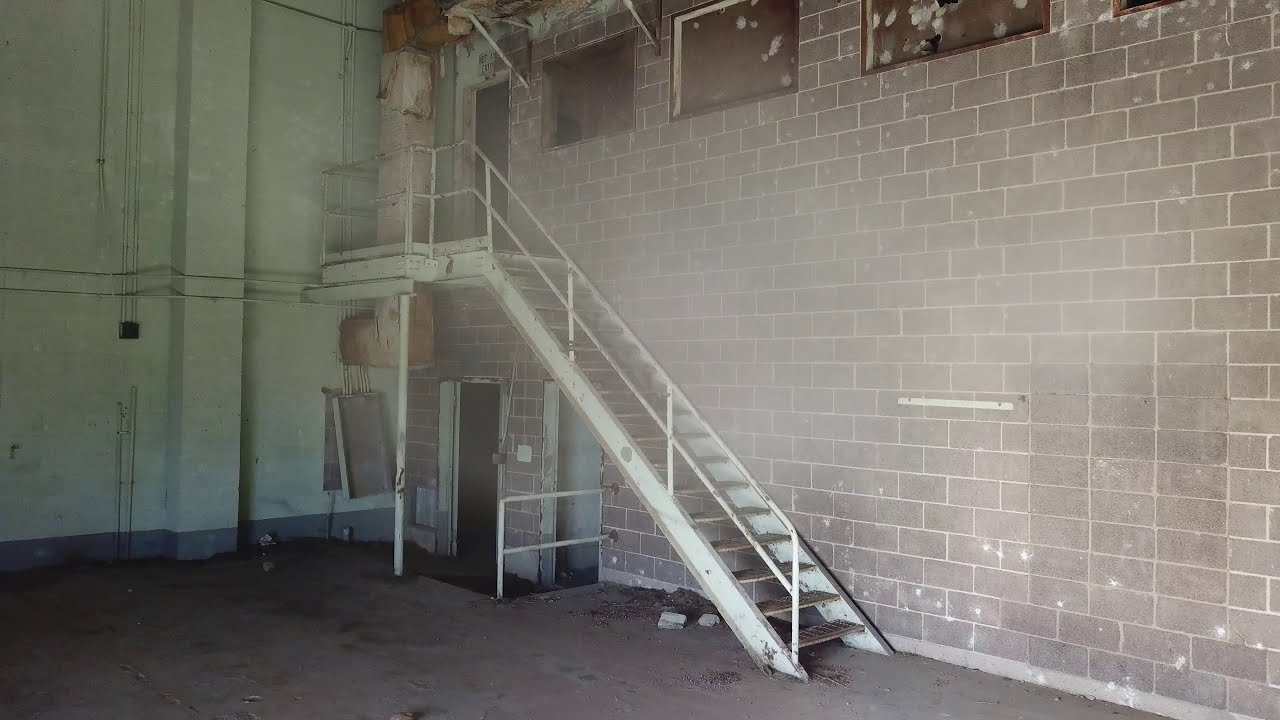The image depicts the interior of a dilapidated industrial building. On the right side, there is a large grey brick wall with sealed rectangular windows on the upper section, which appear to be boarded up. In front of this brick wall is an old, white metal stairwell leading to a closed door on the upper floor, indicating at least two floors in the structure. Below this stairwell are two doorways; one is closed while the other on the right side seems to be open from the inside. The left side of the image features a large, grimy white wall that looks dirty and aged, contrasting with the grey cement floor that shows signs of wear, including visible oil stains. The environment appears dusty and potentially abandoned, with limited natural light illuminating the space, possibly giving it an eerie, haunted atmosphere.